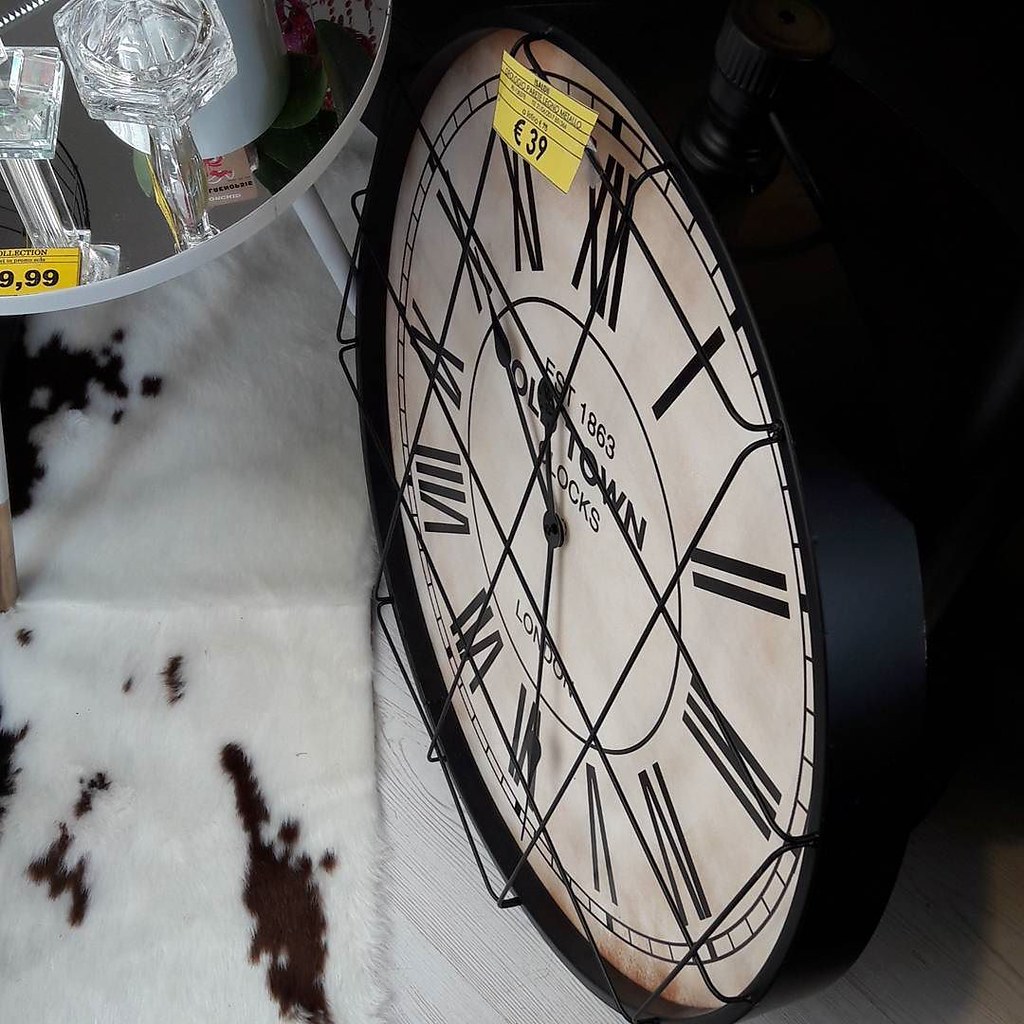The image depicts a close-up view of a large clock prominently on display inside a store. The clock, which is the main focus of the photograph, features black Roman numerals on a white face with black hands, including a second hand. It is housed in a black frame with a small knob at the top resembling that of an old pocket watch. Attached to the top of the clock is a small yellow price tag indicating it costs 39 euros. The clock bears the inscription "Old Town Clocks, Established in 1863, London" towards the bottom of its face. The clock rests on a white fabric with brown spots, possibly resembling a cowhide pattern. In the upper left corner of the image, partially visible, are additional store items including glass candlesticks on display, with another yellow price tag showing the number 9.99 euros. The entire scene conveys a sense of a retail environment with various items on sale.